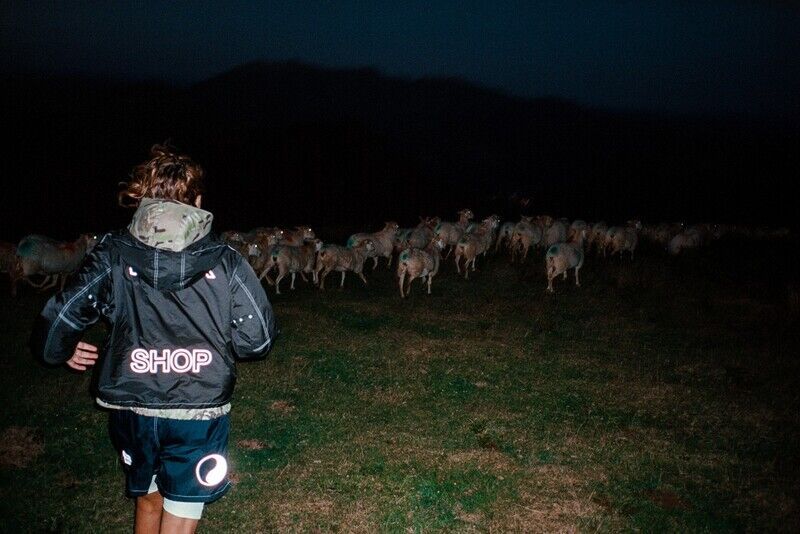In this image taken at night, we see an outdoor field illuminated by a dark sky with a silhouette of mountains in the background. The field is populated by a herd of sheep, around 30-40 in number, which appear to be light-colored with some green paint near their tails, likely from markings. The grass in the field is very short, a tell-tale sign of grazing sheep. 

Towards the left side of the image, a person with brunette hair, possibly tied up in a ponytail, is running after the sheep. This person is wearing a black, reflective, long-sleeved hoodie with the word "SHOP" emblazoned in capital letters across the back. Beneath the hoodie, another hood can be seen poking out, suggesting an additional layered garment. The individual is dressed in black shorts and has light skin. The field of green grass stretches from the middle to the bottom of the image, emphasizing the open nature of the space.